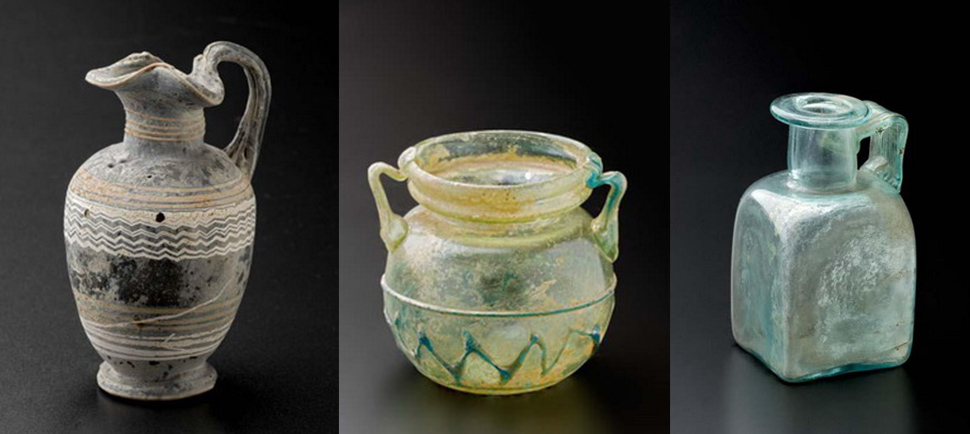This image showcases three antique-looking vessels, each presented against a neutral gray-black background and lined up horizontally. On the left is a very old-looking pitcher made of clay or pottery, featuring a rounded body that narrows to a top with a curved lip. The pitcher is adorned with a zigzag pattern and swirling white lines around its dusty black and tan exterior. Its gnarled handle adds to its ancient charm. 

Moving to the middle, there is a translucent glass container with a greenish tint. Its light brown and yellow hues, combined with traces of worn-off blue squiggly lines, give it an old-world aesthetic. This vessel has two small, irregular handles and a broad open top, with a decorative green X-pattern around the base.

The right-most vessel is a clear small bottle with a bottle-neck and a wide brim. It has a small handle and appears functional, possibly having been used to store medicine. This container, like its counterparts, adds to the historical feel of the collection through its rounded yet somewhat boxy shape and translucent material.